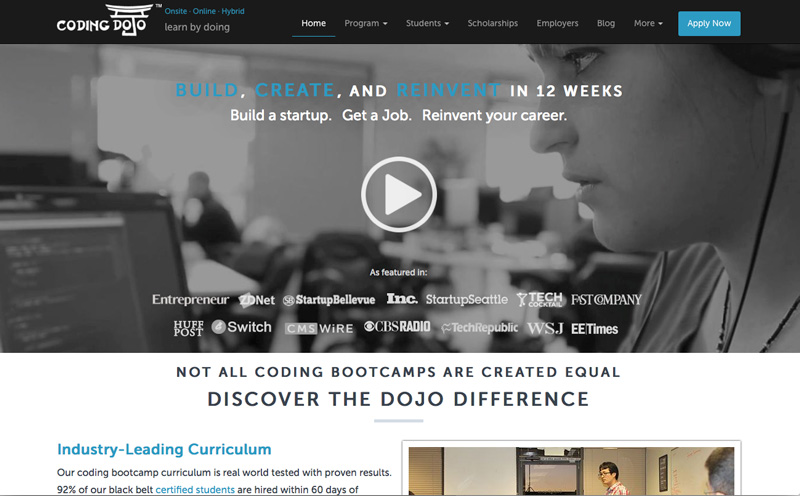This screenshot captures the homepage of the Coding Dojo website, a platform designed for learning coding and computer programming. The top left corner features the website's logo and name, "Coding Dojo," with the 'J' creatively represented by a Japanese Torii gate.

The top navigation bar includes options labeled "Home," "Programs," "Students," "Scholarships," "Employers," "Blog," and a call-to-action blue button that reads "Apply Now." 

Dominating the mid-section of the page is a large, black-and-white photograph of an individual programming on a computer while wearing headphones. Superimposed on the image is an inspiring message: "Build, Create, and Reinvent in 12 Weeks. Build a startup, get a job, reinvent your career." A prominent play button is also present.

Below this section, the logos of various companies that have featured Coding Dojo are displayed. Further down, a bold statement reads: "Not all coding bootcamps are created equal. Discover the Dojo difference." 

The bottom part of the screenshot shows text on the left-hand side, paired with an image on the right-hand side that describes the Coding Dojo's curriculum in greater detail.